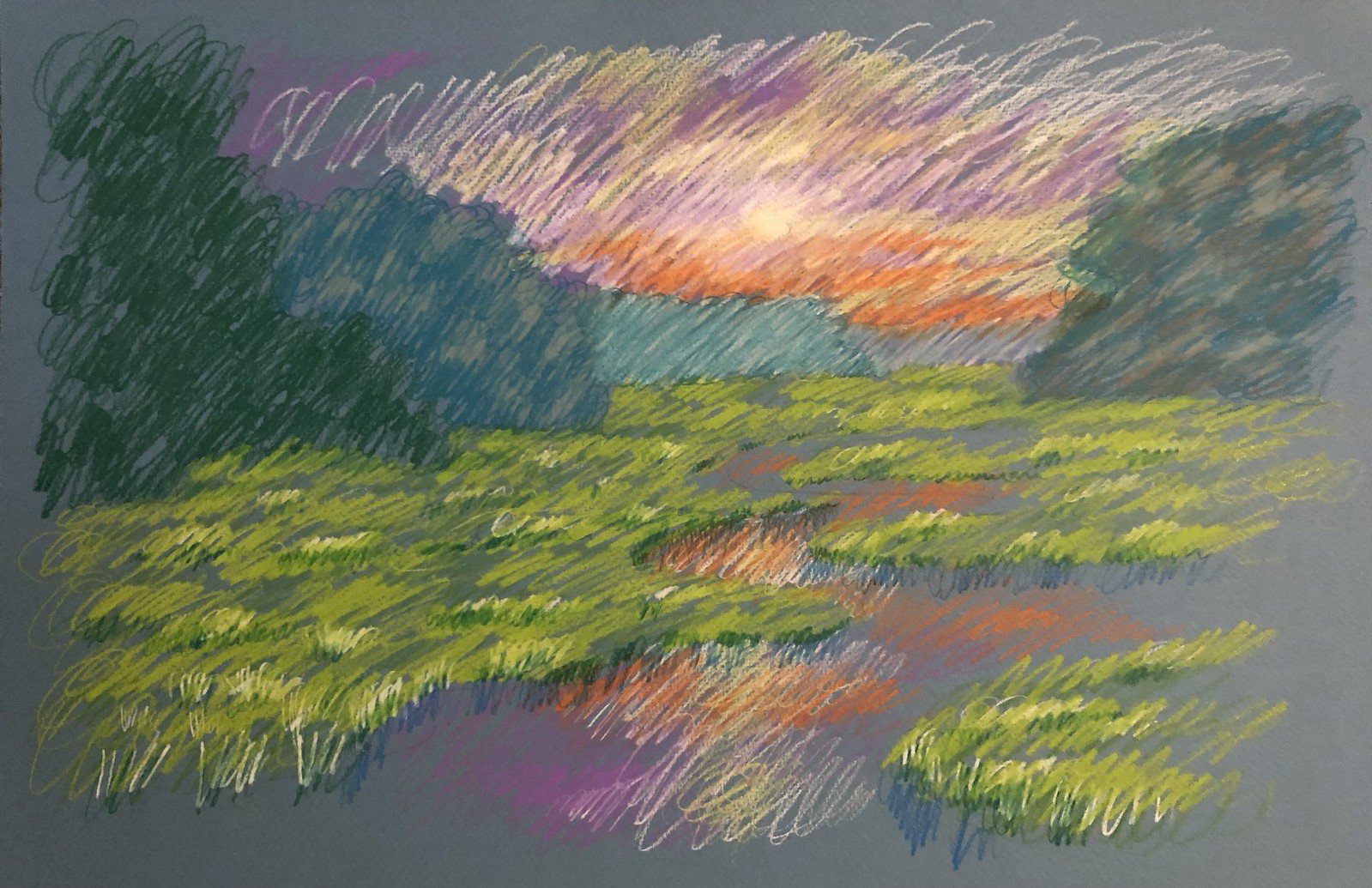This image showcases an abstract piece of artwork depicted on a grey background. The medium used appears to be colored pencils or pastels, creating a texture of swirly, scribbly patterns that blend together to form a cohesive scene. The composition predominantly features a green meadow with light green grass swells occupying the middle ground. Above, a vivid sunset paints the sky with hues of purple, yellow, and orange, clearly highlighting the sun peering through some clouds at the center of the horizon. 

Flanking the meadow, tall trees in dark green and blue shades stand on either side, accompanied by hints of bluish bushes in the background. The scene also includes a suggestion of water or a stream running through the field, reflecting the sunset’s vibrant colors onto the ground. The artwork achieves a delicate balance between the blurred softness of pastel and the detailed strokes of pencil, providing a modern, almost impressionistic, rendition of a serene, natural landscape.